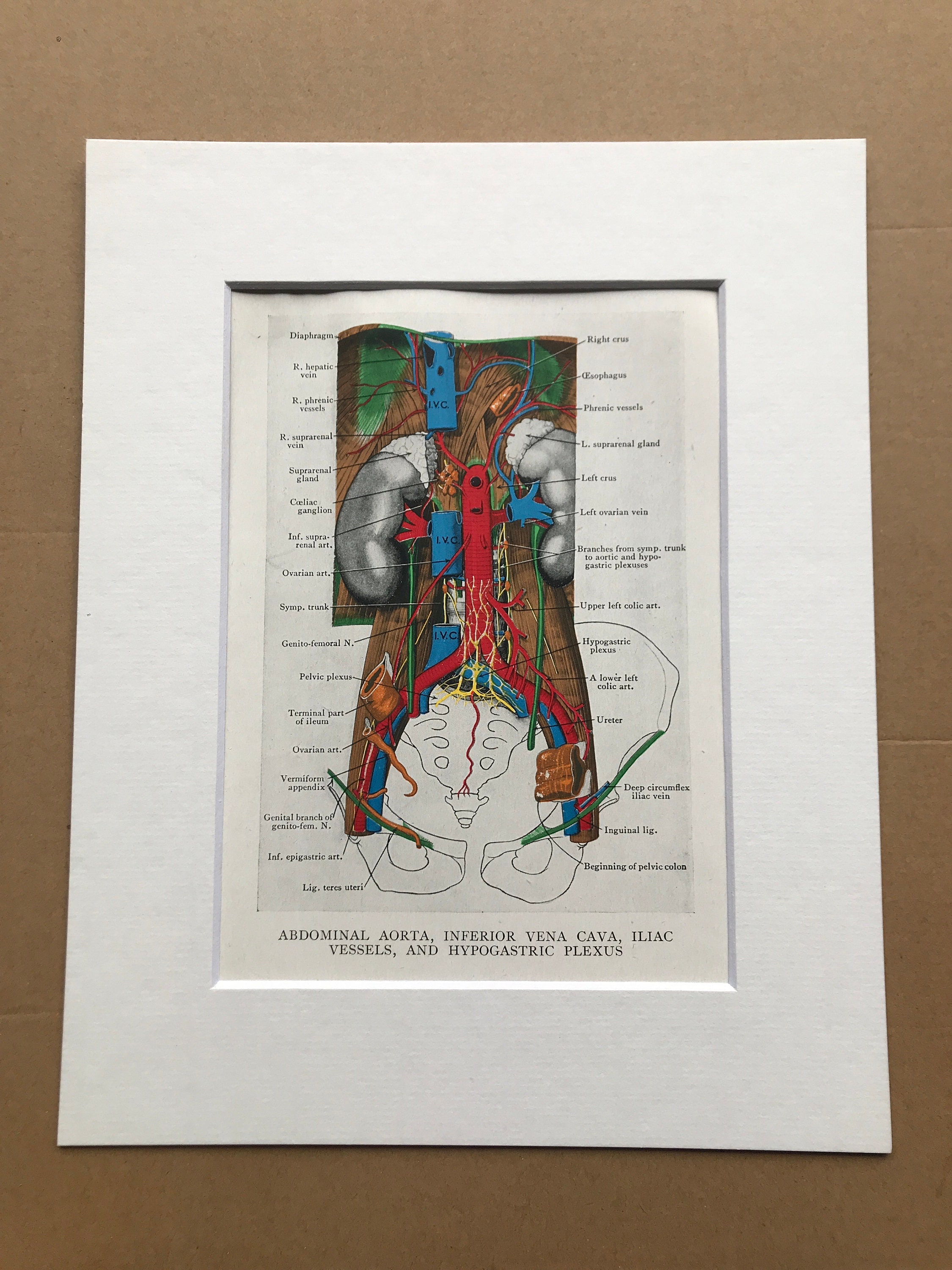This image features a framed medical illustration titled "Abdominal Aorta, Inferior Vena Cava, Iliac Vessels, and Hypogastric Plexus." The diagram, mounted with a paperboard mat, depicts the anatomy of the abdominal and pelvic regions, extending from the diaphragm at the top down to the beginning of the pelvic colon and legs. Key anatomical structures such as the esophagus, left ovarian vein, ovarian artery, pelvic plexus, and celiac ganglion are meticulously labeled. The illustration uses a palette of green, red, blue, gray, and brown to differentiate between the various vessels, nerves, and organs. This detailed diagram showcases the complexity of the human body's internal vascular and nervous systems as understood at the time of its creation.